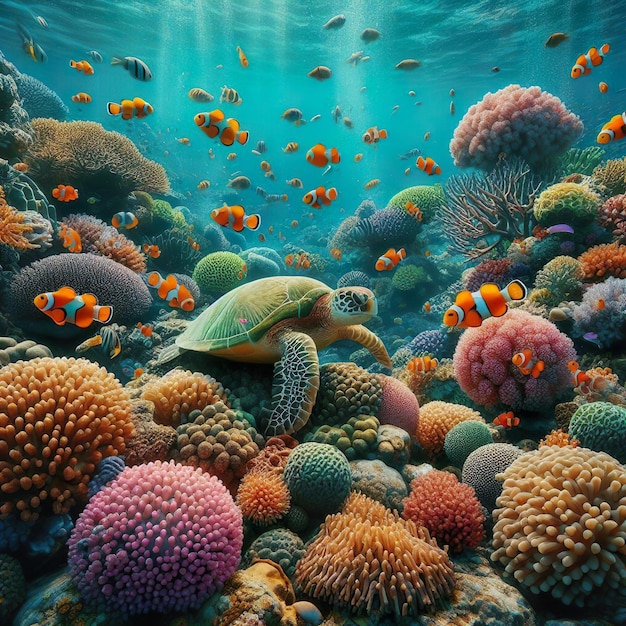This image portrays an enchanting underwater scene, reminiscent of a vibrant coral reef, potentially a photograph taken by a skilled diver. Dominating the center, a majestic turtle with a bright green shell and patterned scales on its head and fins gracefully swims. Surrounding the turtle, a lively assembly of marine life includes numerous mesmerizing clownfish, characterized by their orange, white, and black stripes, alongside other fish adorned in simple black and white hues.

The underwater landscape is rich with diverse flora, featuring sea plants that resemble colorful sea bushes, some with thick, finger-like strands and others with delicate, branch-like forms, creating a varied tapestry of textures. There are also many coral species, ranging in colors from orange, pink, green, and gold to purple, adding to the scene's captivating beauty. Single-cellular organisms like sponges speckle the scene, contributing to the ecosystem's complexity.

Bathed in a serene blue, the water is illuminated by rays of sunlight penetrating from above, casting a magical glow that highlights the vivid colors and the dynamic interplay of light and shadow among the fish and corals. This stunning underwater tableau effectively captures the intricate and colorful life thriving within the coral reef.